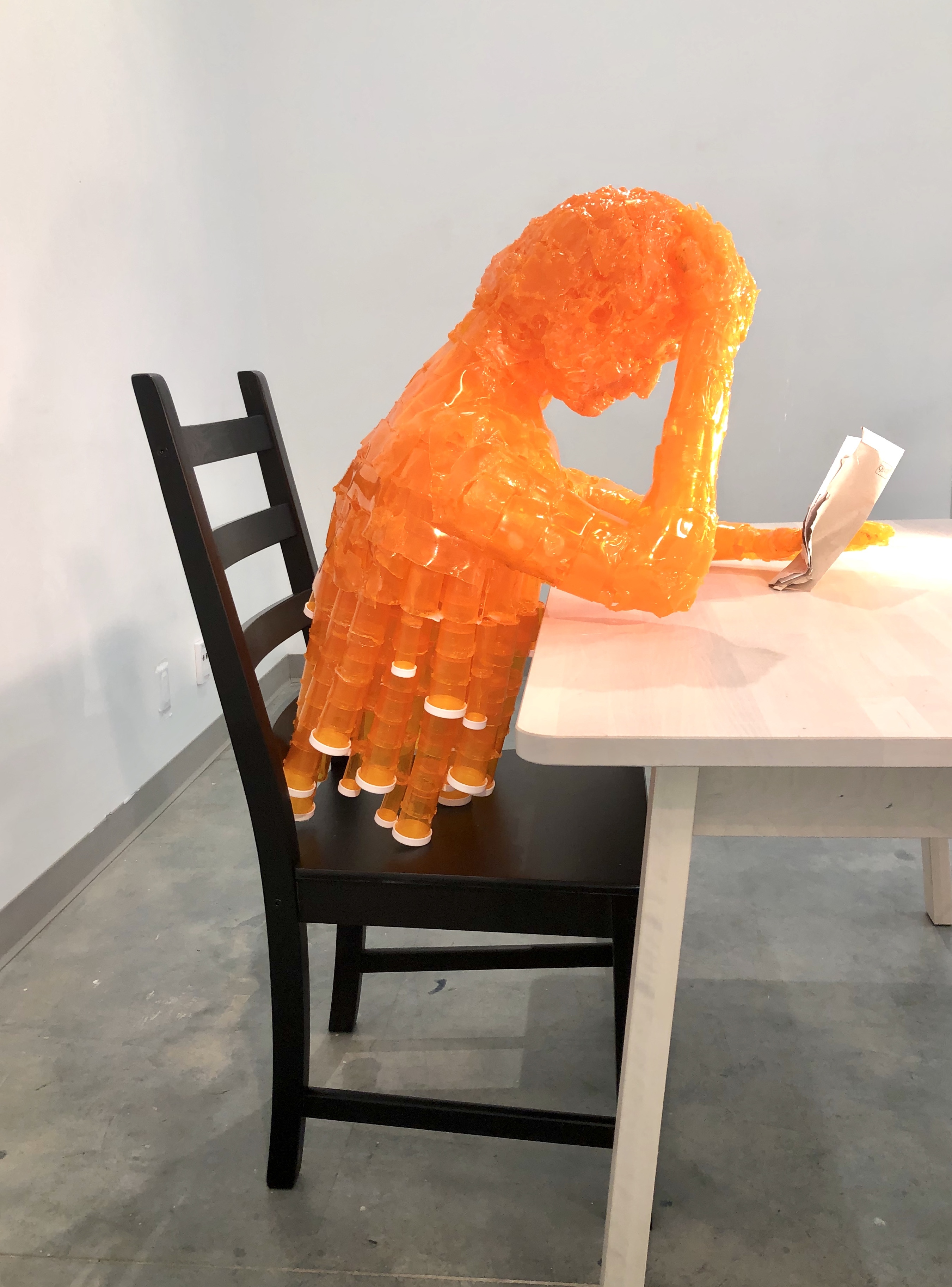The photograph features an art installation situated in a minimalistic room with white walls and a gray concrete floor. At the center of the space is a cream-colored table and a black wooden chair. Seated on the chair is a sculpture resembling the upper torso of a person, seemingly made out of a translucent orange jelly-like substance or possibly prescription bottles. The figure poses with its right hand resting on its head, suggesting a gesture of concentration or contemplation, while the left hand holds a piece of paper or book that the figure appears to be intently reading. The installation, with its strikingly lifelike posture, evokes a scene of deep reflection and thought.